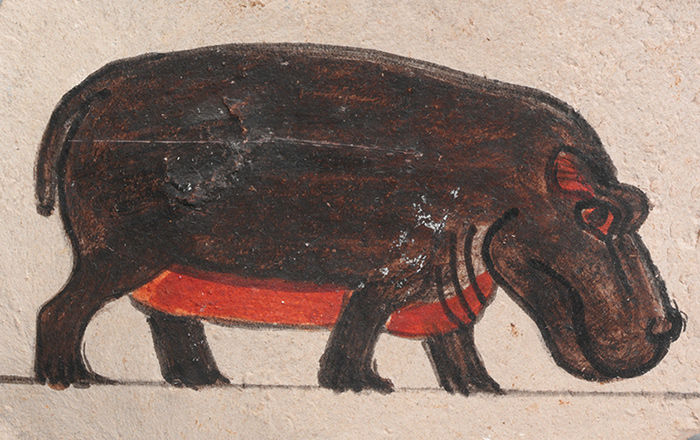This is a crayon drawing of a large hippopotamus depicted in a dark brown hue with distinct features. The hippo has striking red eyes with black pupils and a red underbelly, adding contrast to its overall dark coloring. Some white spots can also be observed along its body. The animal is positioned centrally on the light tan paper, with its head bending down towards the ground, giving the impression it might be grazing. The hippo is oriented facing right, showing only its right side, with a small, stumpy tail visible in the back. The plain backdrop and clear quality of the image, enhanced by natural lighting, make the details of the hippopotamus stand out. There are no additional animals, text, numbers, or signatures in the image, focusing attention solely on the meticulously colored hippopotamus.